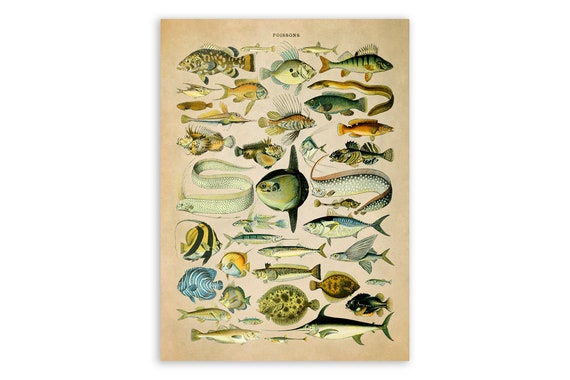The image is a detailed botanical poster of various fish species. The rectangular poster features an aged cream-colored background, which is noticeably darker at the corners, giving it a vintage look. The top of the poster has a small, partially unreadable text, presumably indicating that the poster's subject is fish, possibly labeled "poissons" in French. The fish are intricately hand-drawn in a clustered formation, with over 30 species represented, each illustrated to reflect their natural colors. 

Some of the identifiable species include eels, sunfish, catfish, swordfish, flounder, pufferfish, marlin, angelfish, and tigerfish. The layout consists of fish positioned in loosely aligned rows, ranging from four to five fish per row, although not perfectly symmetrical. Specific details highlight individual fish, such as a brown, thickset fish with lighter dots, various yellow and blue exotic species, green and brown eels, and other uniquely patterned fish like a tigerfish and a marlin. 

The illustration style emphasizes the retro aesthetic of the poster, making it not just an informative chart for fish identification, but also an artistic display of marine life. The diverse array of species, coupled with the meticulous hand-drawn quality, captures the beauty and variety of oceanic fish in an engagingly detailed and visually appealing manner.